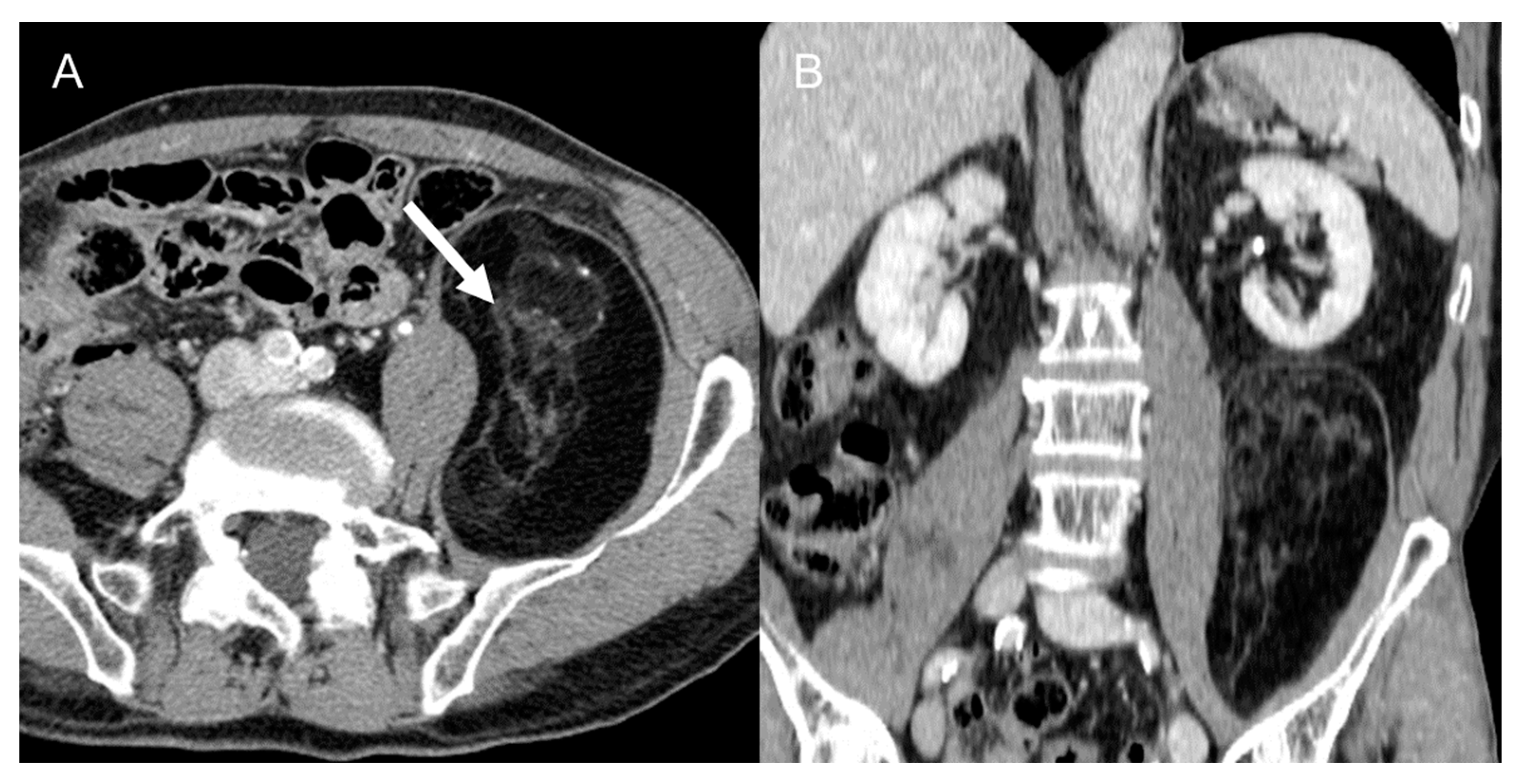This horizontally aligned, black and white image consists of two side-by-side x-ray sections, labeled A and B in the upper left corners of each respective image. Both sections are overlaid on a black background and are seemingly related to the human body's internal organs.

In section A, situated on the left, there’s a solid black background with the letter A in the upper corner. This section highlights a kidney-shaped object, indicated by a white arrow pointing to a grayed area amidst an irregularly shaped oval black region. Surrounding this are white lines and a porous area on the top, all encased within a thin gray outline.

Section B, on the right, also starts with a black background mostly visible at the top and contains the letter B in the upper left corner. This section is more complex, featuring large gray-shaded areas interspersed with highlighted white regions. Centrally located are small, rectangular bordered areas, likely representing a close-up view. More porous sections appear on the left and bottom, and despite some variations in interpretation, it appears to depict a different angle focusing on the kidneys. The kidney on the left is intact, while the kidney on the right seems partially missing. This section may also display other parts like the spine and potentially the lungs.